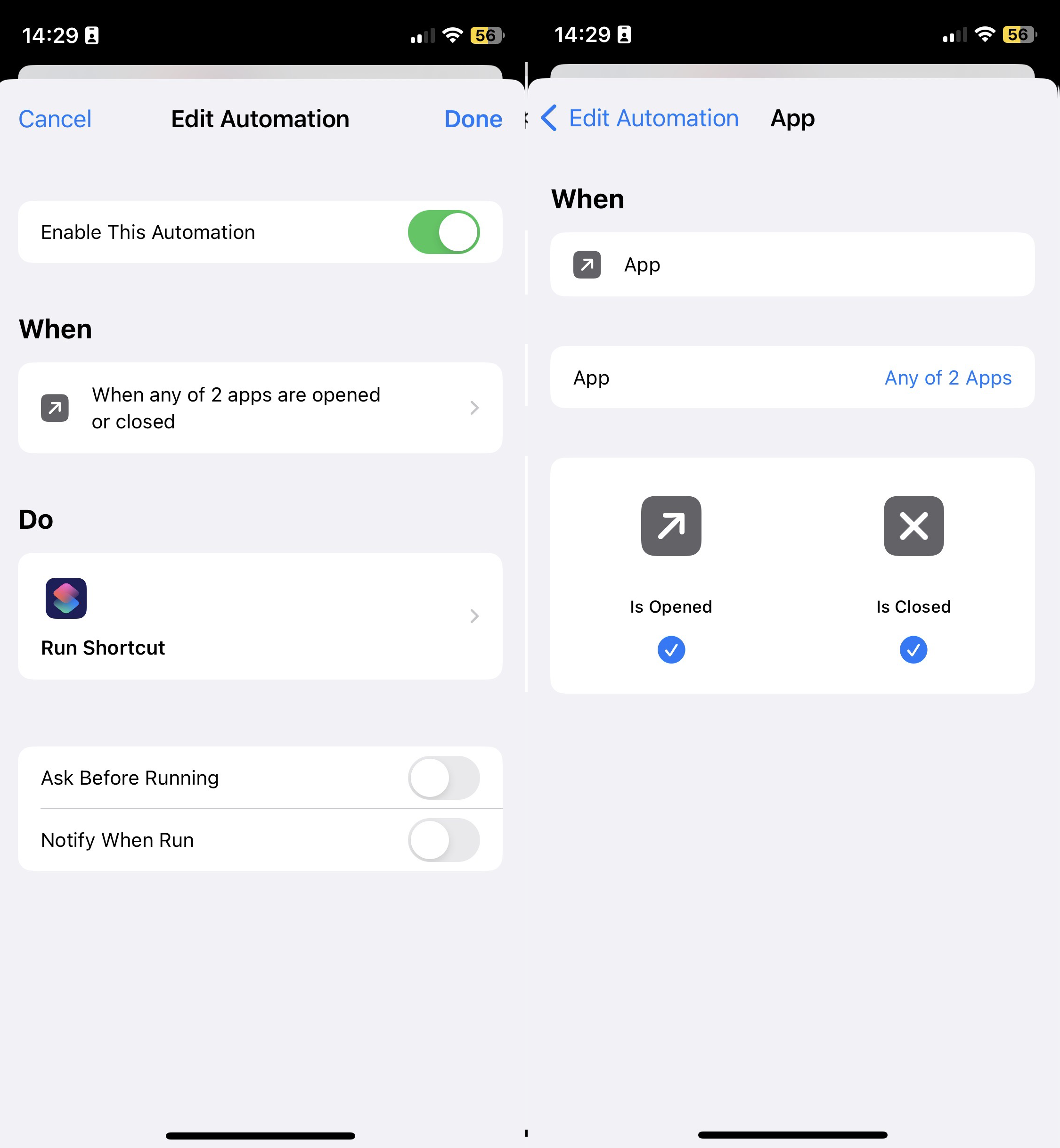The image shows a detailed view of the "Edit Automation" settings on an iPhone. On the left side, the first window is titled "Edit Automation." At the top, there are "Cancel" and "Done" buttons. Beneath that, a toggle labeled "Enable This Automation" is switched on, indicated by a green button. Under the section labeled "When," it states, "When any of two apps are opened or closed," with an arrow button next to it. Below this, the action specified is "Run Shortcut." Further options listed are "Ask Before Running" and "Notify When Running," neither of which are selected.

On the right side, the second window shows more details linked to the previous settings. The title "App" appears next to "Edit Automation" at the top. It begins with "When App," followed by an arrow indicator. Beneath this, "App any of two apps" is highlighted in blue text. Below, it specifies the conditions "Is Opened" and "Is Closed," both marked with blue backgrounds and a small white checkmark in their centers.

The overall color theme is gray, blue, and white, consistent with the standard iPhone interface design, except for the icons that retain their usual colors.